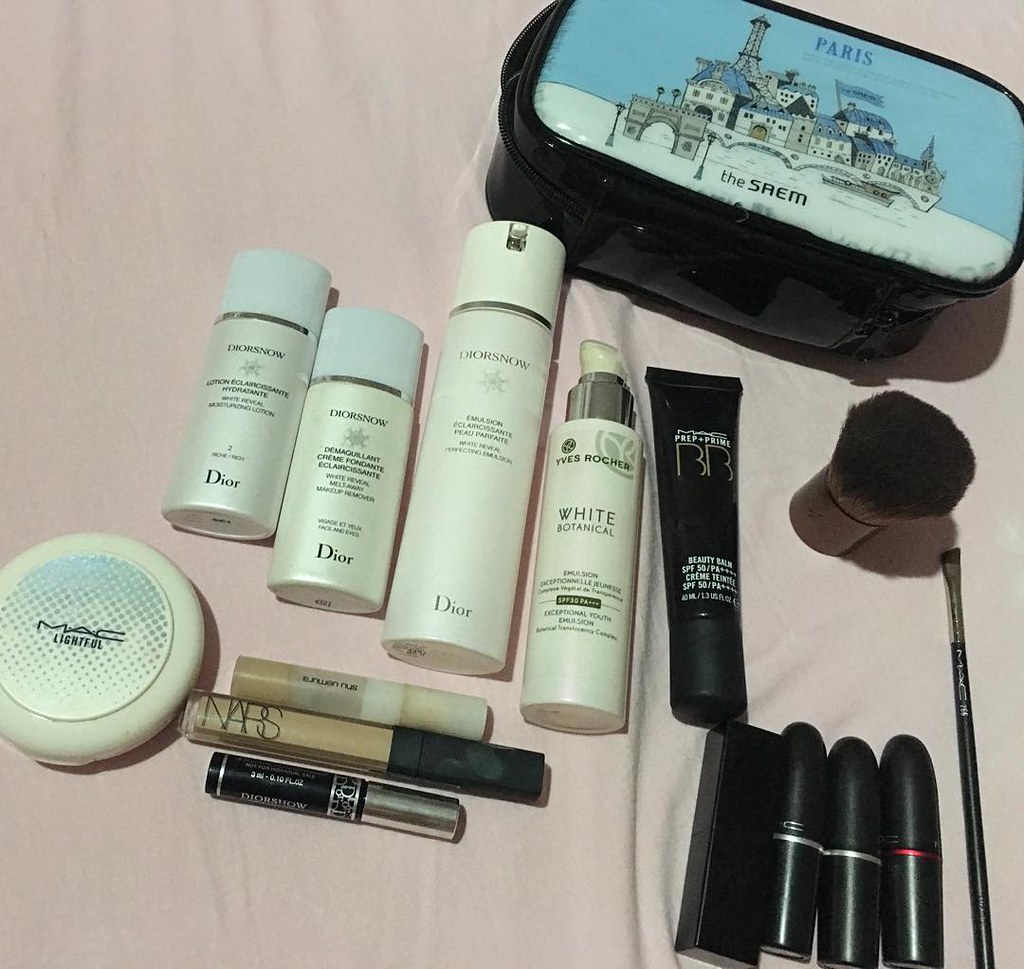The color photograph features a pink tablecloth adorned with an assortment of makeup items. In the upper right corner, there is a black makeup bag with a colorful illustration depicting the Paris skyline, showcasing iconic landmarks like the Eiffel Tower and various architectural buildings in shades of blue and white. Below the bag, different makeup products are neatly arranged. These include a brown brush, multiple shades of lipsticks, and a black tube labeled "BB." To the left, there are several white pump bottles from Dior, accented with green and white labels. Nearby lies a concealer puff pad, a tube of mascara, and a thin eyeliner brush. Each item is meticulously placed, creating a visually appealing and organized display.